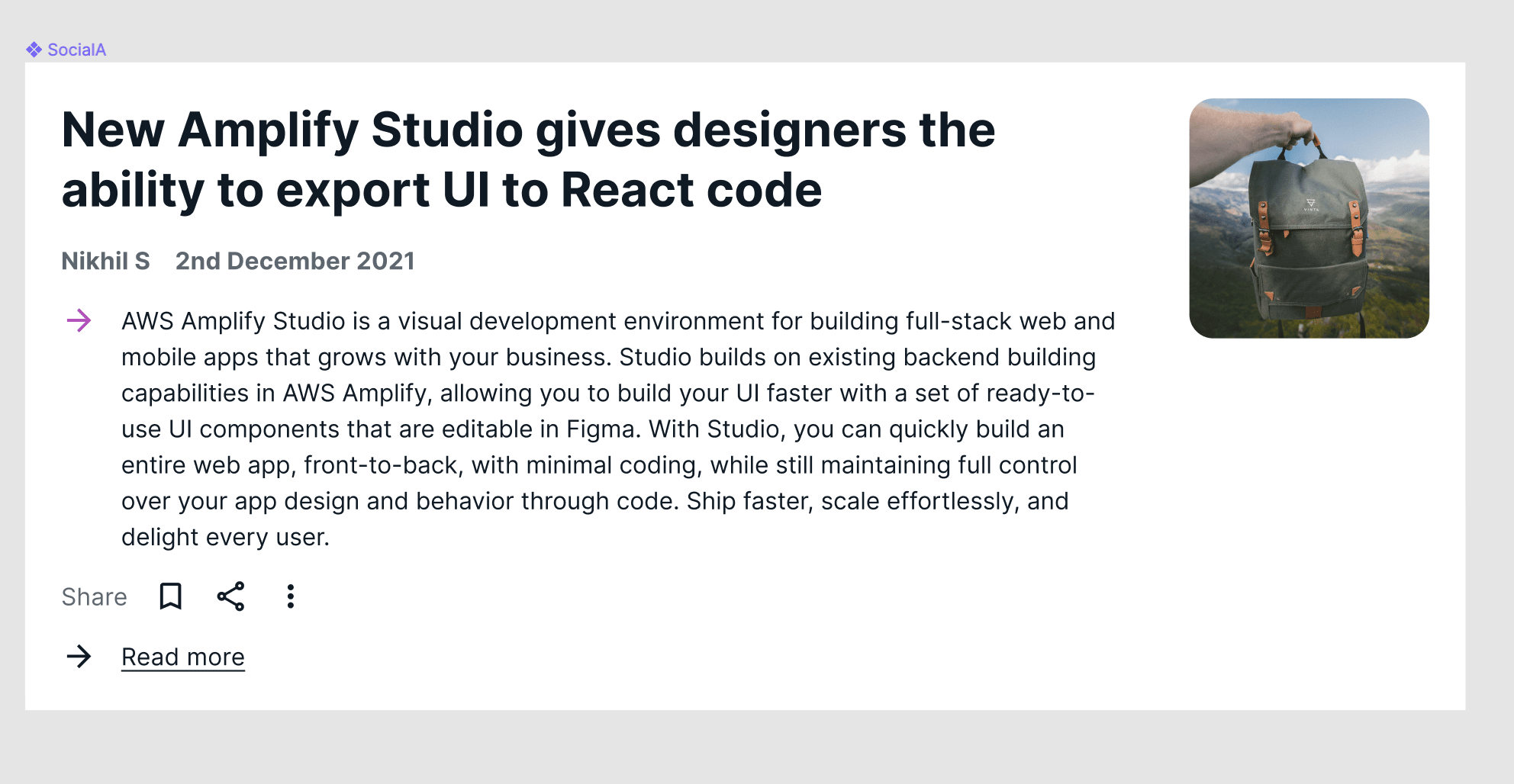This is a landscape-oriented photo capturing a section of a website displaying a news article or blog post. The layout prominently features a white content box centered within a thin grayish border. In the top left corner of this gray border, there is a blue or purple diamond-shaped icon accompanied by the text "Social A" in purple font.

The white content box contains several elements. At the top, there's a bold, black headline stating "New Amplify Studio gives designers the ability to export UI to React code." To the right of the headline is a square-shaped image with rounded edges showing a backpack being held by an individual's arm against a scenic backdrop of sky and mountains.

Below the headline and image, on the left side, is the author's name, "Nikhil S," alongside the publication date, "2nd December 2021." Directly beneath this information is a pink right-facing arrow leading into a body of text, presumably the article's introduction or main content. Below the text, there are various interactive elements, including links, share buttons, a bookmark option, and an ellipsis menu. At the very bottom, a black right-facing arrow accompanies a link labeled "read more."

The overall impression is that of a tech blog, possibly detailing new features or tools relevant to designers and developers, showcased by an author sharing their insights or news.